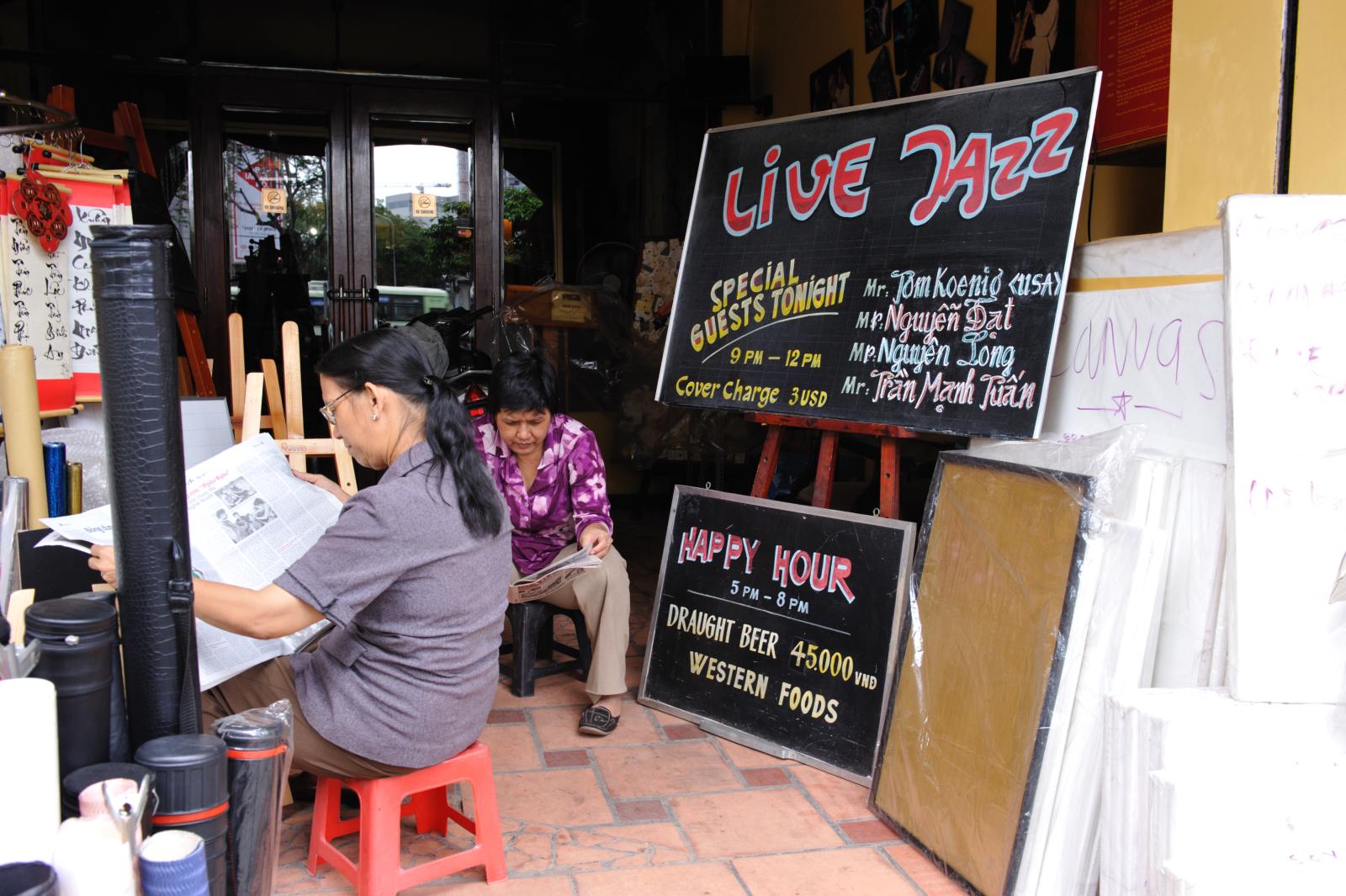In this detailed photograph taken during daylight, we see the storefront of a restaurant, possibly outdoors on a tiled floor. The scene is centered around two women of Asian descent, both absorbed in reading newspapers while seated on plastic stools—one black and one red—near the middle of the image. The woman on the left is dressed in a purple floral shirt and khaki pants. 

To the left side of the image, cylindrical containers, presumably scroll cases, are displayed along with wooden easels for sale. Above these are several banners with red headers and footers and Asian script, indicating they are also for sale.

On the right side of the image is a prominent black sign with a silver outline, propped on a wooden easel. This sign announces "Live Jazz" in red letters with a blue outline, "Special Guests Tonight 9 p.m. to 12 p.m." in yellow, and lists performer names: Mr. Tom Koenig (USA), Mr. Nguyen Dat, Mr. Nguyen Long, and Mr. Tran Manchuan. Beneath this main sign, another smaller black sign with a silver outline reads: "Happy Hour" in red, "5 p.m. to 8 p.m." in white, "Draft Beer 45,000 VND," and "Western Foods" in yellow.

The back of the area features closed wooden doors with glass panels, contributing to the storefront appearance. Mixed with these elaborate details are vibrant splashes of color throughout the image, including shades of black, red, light blue, yellow, pink, and orange, alongside different shades of gray.